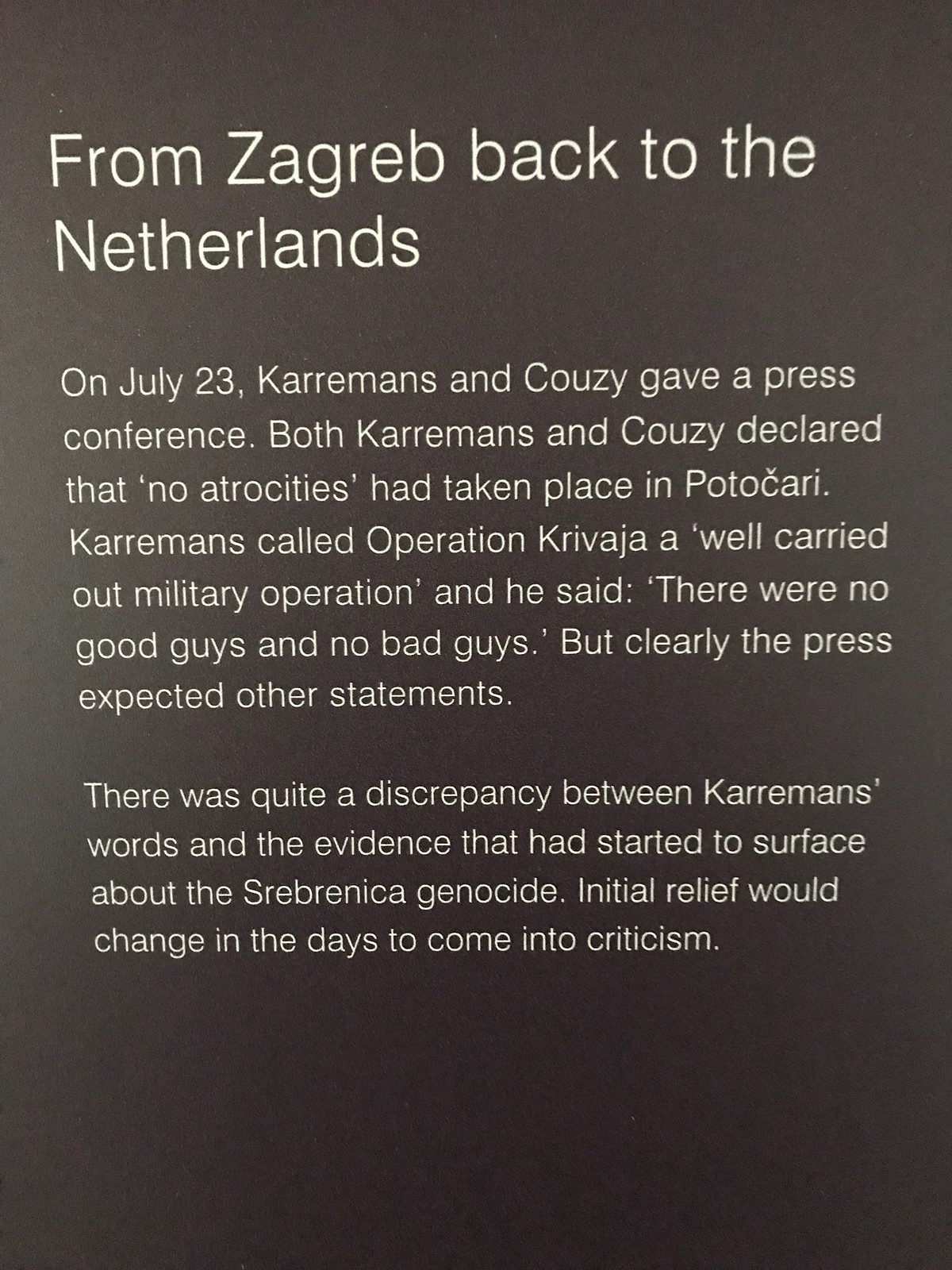The image features a slide with a light black background and white text. At the top, in bold, it reads: "From Zagreb back to the Netherlands." Below, in regular white text, a paragraph details the events of a press conference held on July 23, where Karamans and Kossi (sometimes referred to as Kuzi or Kouzi) declared that no atrocities had taken place in Potocari. Karamans described Operation Krivazha (possibly mentioned as Operation Kariba or Kravia) as a well-carried-out military operation, emphasizing that there were no "good guys" or "bad guys," contrasting the press's expectations for their statements. A second paragraph highlights a discrepancy between Karaman's assertions and emerging evidence of the Srebrenica genocide, predicting that initial relief would soon turn into criticism as more information surfaced.